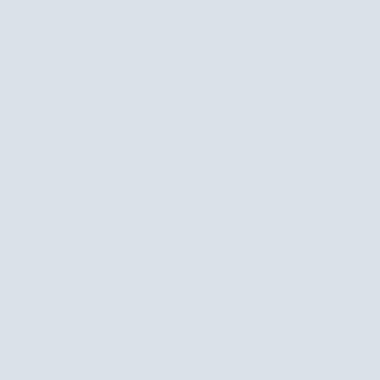The intended photograph failed to load, resulting in the display of a plain gray square. There is no image to review or describe due to this technical issue. We apologize for the inconvenience and appreciate your understanding.